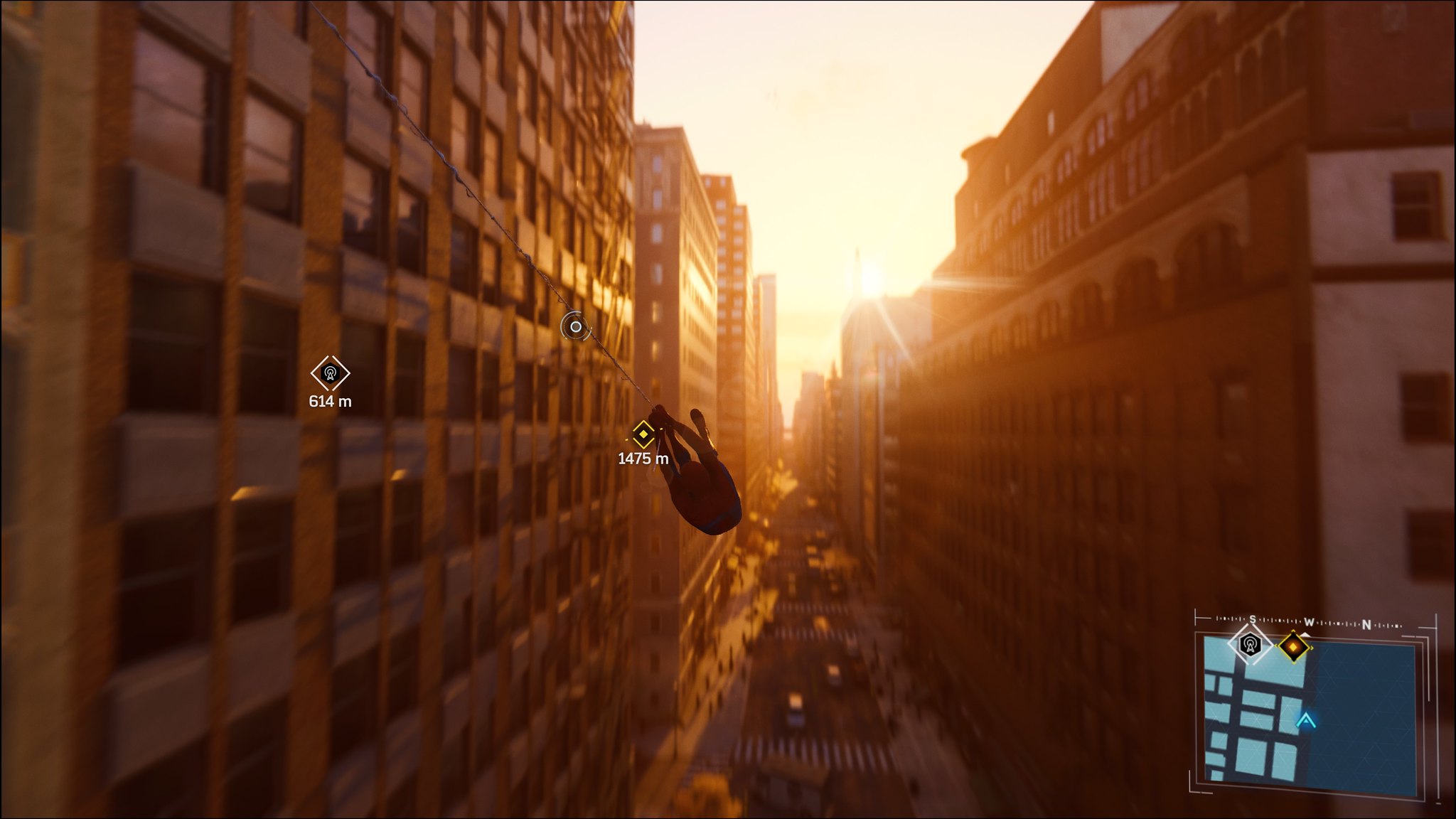This is a detailed, computer-generated screenshot from a Spider-Man video game. The image is in landscape orientation and vividly colored, boasting an overly perfect appearance suggesting it isn't a photograph. The scene captures Spider-Man swinging through a bustling urban cityscape, framed by towering high-rises. The perspective is set halfway up these buildings, looking down upon a gridded street teeming with cars and city life below. In the distance, sunlight bathes the horizon in a warm, yellow-orange hue, indicating it is either sunrise or sunset, most likely sunset.

Prominent in the foreground is Spider-Man, ensconced in shadows as he navigates the air between buildings on a web. He appears to be heading towards a map marker, with two visible markers: one at 1475 meters and another at 614 meters. These markers are yellow diamond shapes with corresponding distances in white text. On the bottom right of the screen, a detailed mini-map displays Spider-Man's current location in the city, bordered with small white lines and additional markings. The overall composition of the image, combined with the evident details, underlines its origin as a high-fidelity video game representation rather than a real photograph.